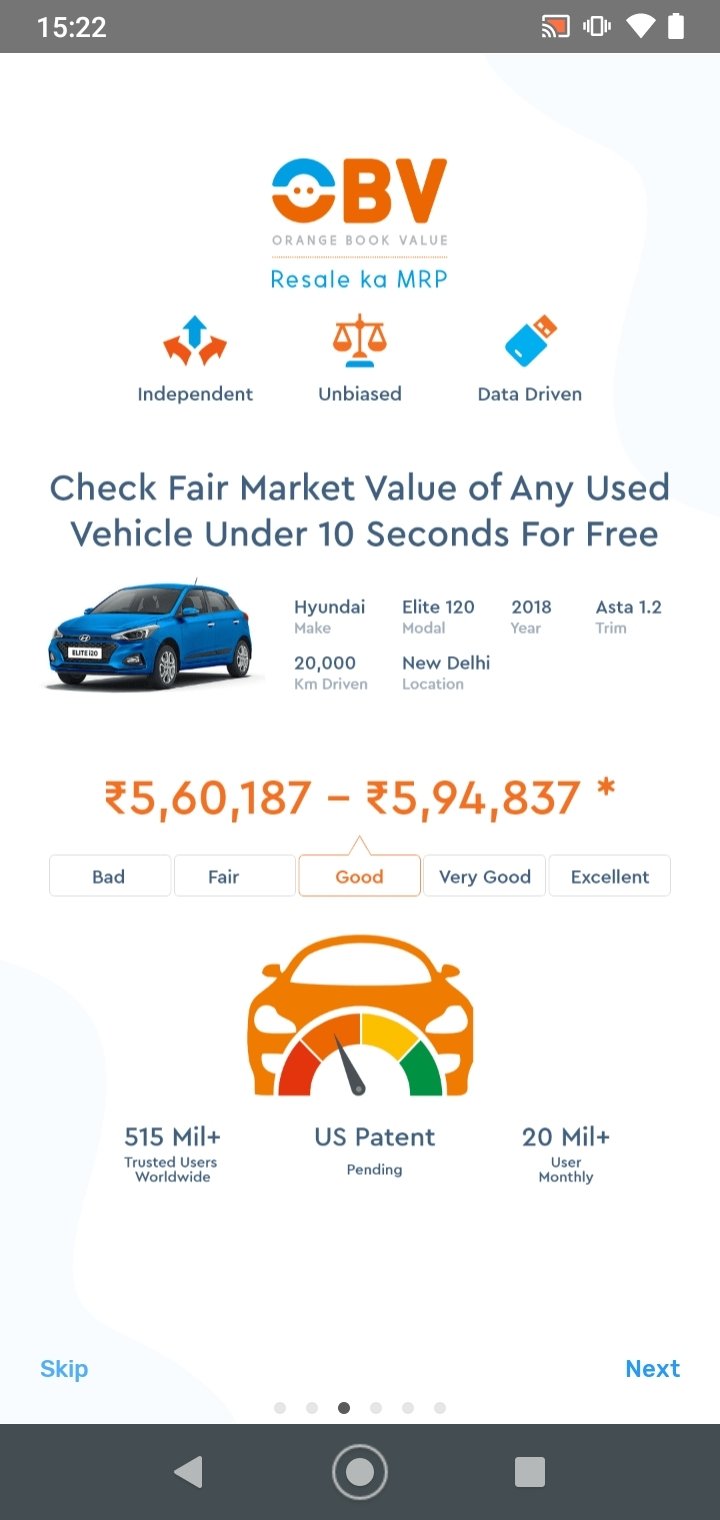**Image Caption:**

A vertically oriented screenshot from an Android phone displaying a car valuation application. The image shows the status bar at the top indicating the time "15:22," Wi-Fi and cellular signal strengths, battery level, and an unrecognized icon. 

The main screen is predominantly white, containing various colorful texts and a small image of a blue Hyundai Elite i20, model year 2018. At the top, there is an unclear abbreviation "OBV," which might stand for "Orange Book Value" or another term. Below it, an incorrect or garbled word "KAMRP" appears where some readable text is expected.

The app provides the resale value of the vehicle in Indian Rupees, listing it between ₹5,60,187 and ₹5,94,837, the latter accompanied by an asterisk with no further explanation provided. The user interface includes a description stating, "Check fair market value of any used vehicle under 10 seconds for free."

There is a rating system below the vehicle value, with categories: Bad, Fair, Good, Very Good, and Excellent. The user's selection is "Good," aligning the estimated value in the "Good" category. A stylized graphic mimicking a speedometer with red, orange, yellow, and green segments shows an arrow pointing to the orange segment, representing the "Good" condition.

Additional text at the bottom mentions "515 MIL+," "U.S. Patent Pending," and "20 MIL+," though their significance is unclear. Finally, options to "Skip" or proceed to the "Next" vehicle are provided at the bottom of the screen for further navigation.

***End of Caption***